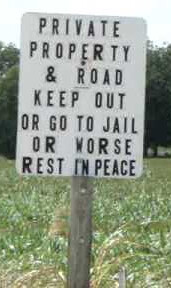This photograph captures a foreboding private property sign anchored on a weathered, greyish wooden post, situated amidst a green field. The large white sign features bold black text that reads: "Private Property and Road. Keep Out or Go to Jail or Worse, Rest in Peace," emphasizing the property owner's strict and potentially lethal stance on trespassing. Surrounding the sign is a stretch of green grass, interspersed with occasional brown patches, suggesting untamed and somewhat neglected vegetation. In the background, a dense array of towering, dark green trees forms a natural barrier, and above, a sky of light blue mixed with white completes the scene, adding a serene yet stark contrast to the menacing warning below.